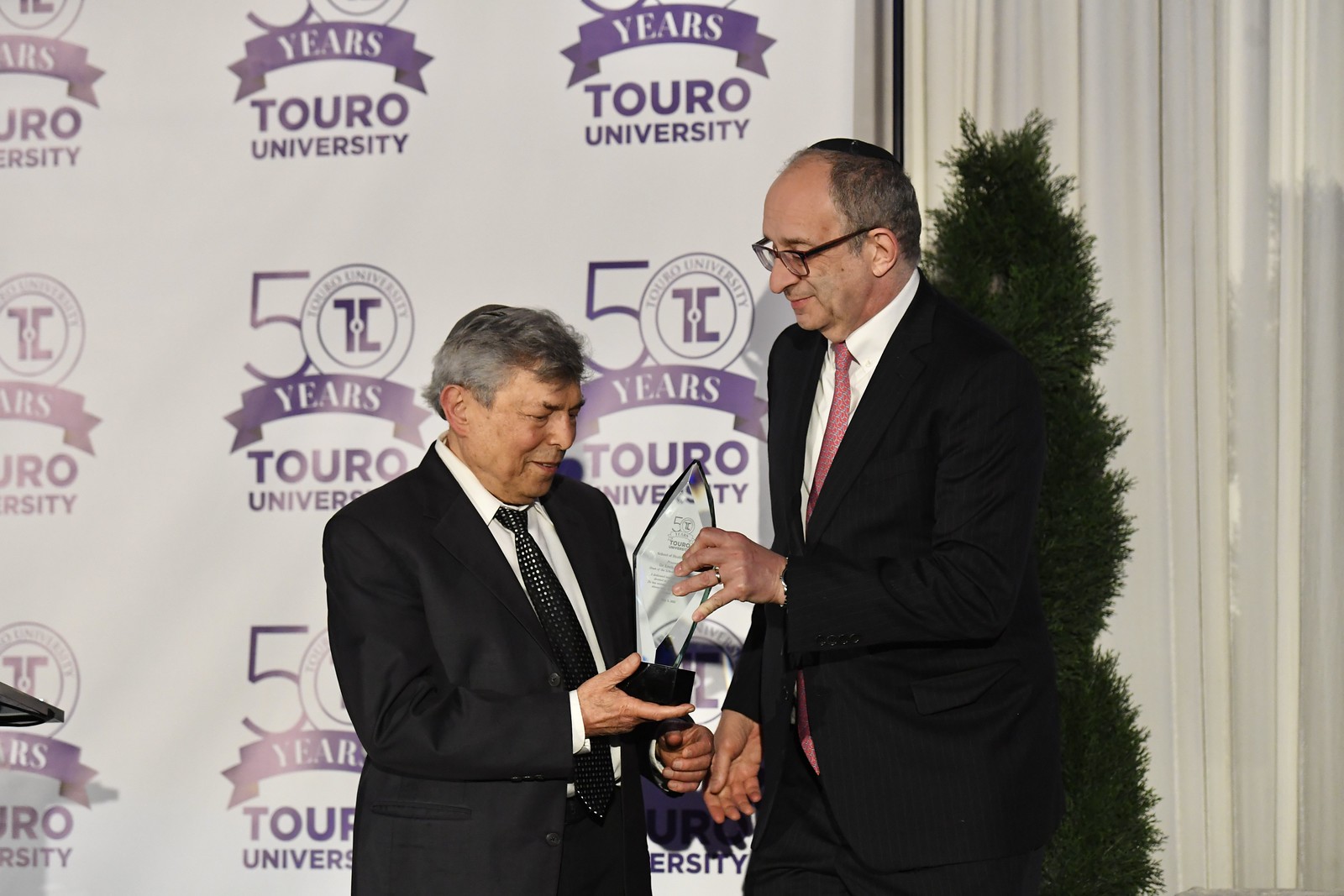The photograph captures an indoor setting featuring two older men at what appears to be an award presentation. Both are dressed in black suits with white shirts, but their ties differ: the man on the left wears a black tie with white dots, while the man on the right, who also wears glasses, sports a pink tie with dots. The man on the left is receiving the award, holding its base with one hand as he looks at it intently, while the man on the right supports the top of the award with his fingers. The award itself is made of glass and is quite tall and ornate. The background showcases a large poster with multiple repetitions of the Touro University logo and the text "50 Years Touro University" in purple set against a white background. To the right of the poster, there's a small green plant and a white curtain behind it.